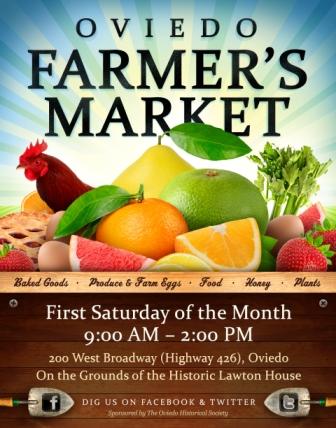The vibrant and colorful poster advertises the Oviedo Farmers Market, prominently featuring a rooster perched among a plethora of fruits and vegetables, including oranges, pears, celery, lemons, limes, strawberries, a cut watermelon, and apple pie. The poster includes text in various colors: "Oviedo Farmers Market" is boldly displayed in black across the top against a backdrop of sun rays. Italicized text in the middle highlights the offerings such as baked goods, produce, farm eggs, food, honey, and plants. The bottom section of the poster, set against a brown background, details the event specifics in white lettering: "First Saturday of the month, 9 a.m. to 2 p.m., 200 West Broadway Highway 426, Oviedo, on the grounds of the historic Lawton House." Additional text encourages viewers to "Dig us on Facebook and Twitter," accompanied by garden spade icons with the respective social media symbols. The poster, sponsored by the Oviedo Historical Society, effectively captures the essence of the market with its engaging imagery and comprehensive information.